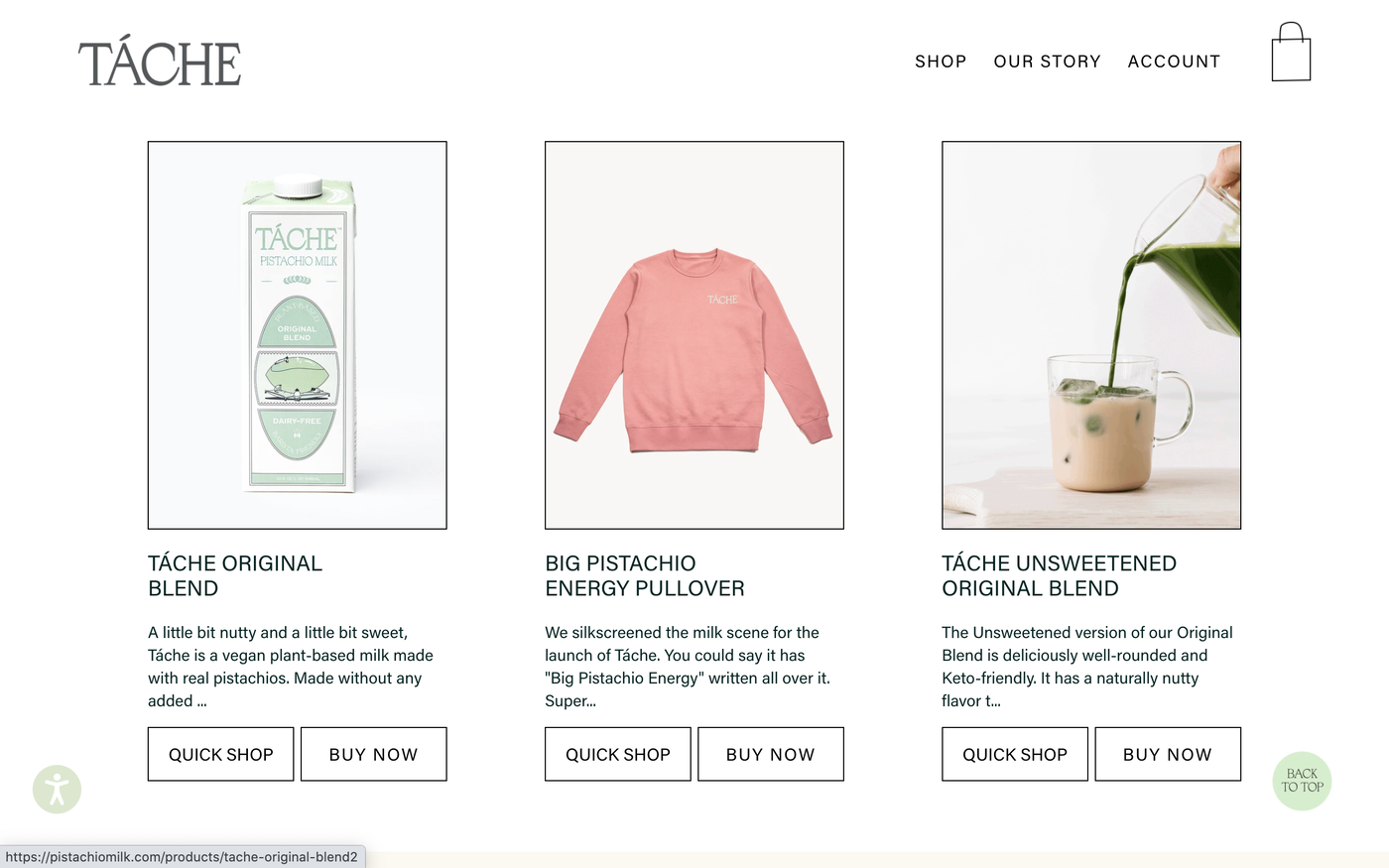The image is a meticulously designed webpage from a company named TACHE, set against a pristine white background. On the right-hand side of the webpage, there are navigation options including "Shop," "Our Story," and "Account," accompanied by an icon of a shopping bag. 

The main section of the webpage features three distinct product offerings:

1. **TASH Original Blend**: This section boasts a tagline that reads "A little bit nutty and a little bit sweet." Described as a vegan, plant-based milk made with real pistachios and free from any added sugars, it provides options for "Quick Shop" and "Buy Now."

2. **Big Pistachio Energy Pullover**: Centrally situated, this product is highlighted with the title "Big Pistachio Energy Pullover," shown in pink. The description mentions that the design was silk-screened to celebrate the launch of TASH, encapsulating the vibrant energy of pistachios. It also offers "Quick Shop" and "Buy Now" options.

3. **TASH Unsweetened Original Blend**: The final product showcased is the "TASH Unsweetened Original Blend," noted for its well-rounded, naturally nutty flavor that is also keto-friendly. The image features someone pouring this green pistachio milk into an iced coffee within a clear glass. Similar purchasing options include "Quick Shop" and "Buy Now."

The overall layout and aesthetic are clean, with an additional visual featuring a green-themed image displayed on both the bottom right and left corners of the page.